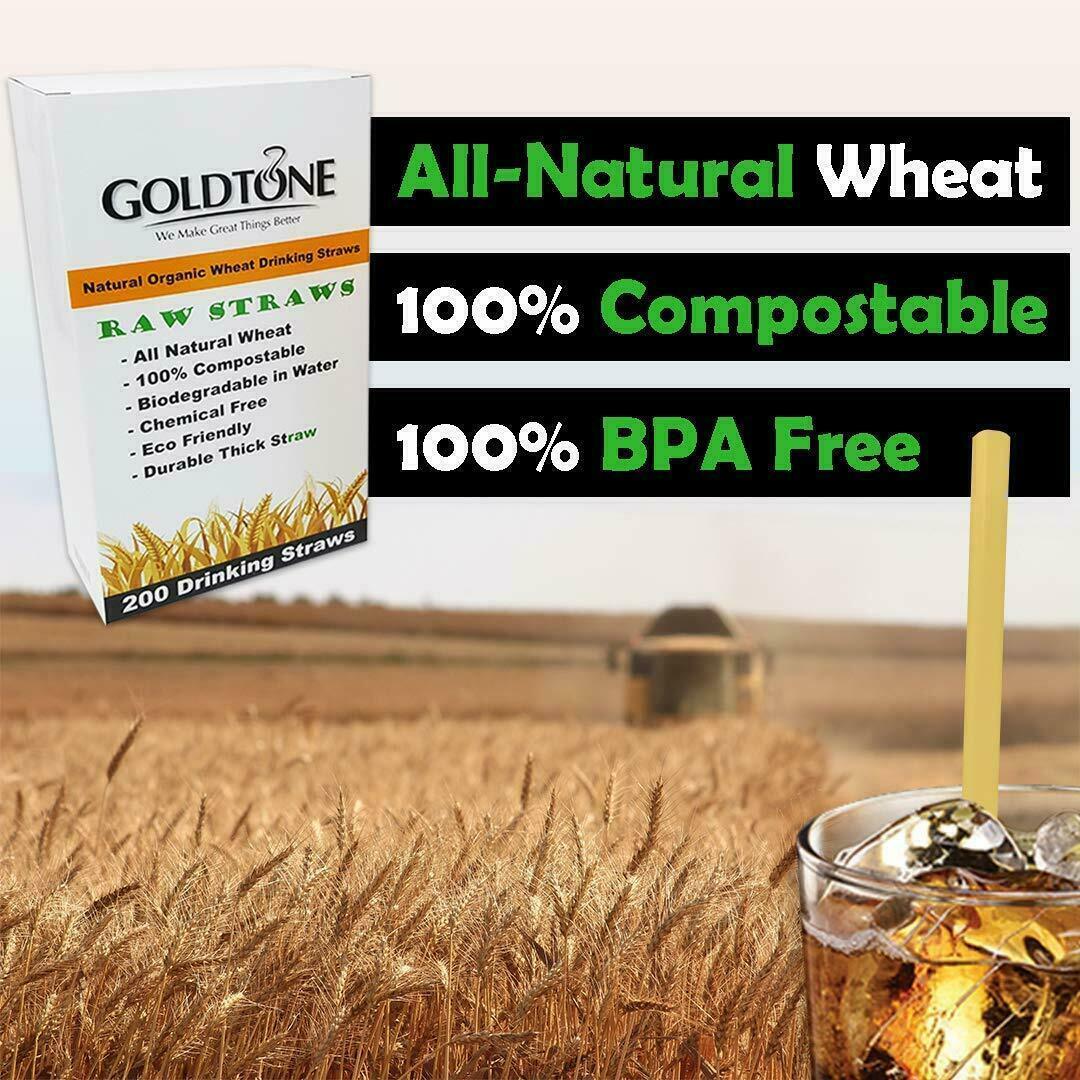The image showcases an outdoor scene with a whimsical sky gradient transitioning from light pink at the top to light gray at the bottom. Dominated by a lush wheat field, the background also features a distant, slightly blurry structure, possibly a combine harvester. A refreshing iced beverage in a glass jar, complete with a yellow straw made from natural organic wheat, peeks into the lower right corner, enhancing the rural aesthetic.

Prominently positioned in the upper left, a white box outlines the product being advertised: "Gold Tone Natural Organic Wheat Drinking Straws." This detailed advertisement highlights the eco-friendly attributes of the straws, describing them as "All-Natural Wheat, 100% Compostable, Biodegradable in Water, Chemical-Free, Eco-Friendly, Durable, Thick Straw." The packaging indicates that each box contains 200 drinking straws.

Additionally, the ad emphasizes the environmental benefits with text in green and black on three black backgrounds: "All Natural Wheat, 100% Compostable, 100% BPA Free." The overarching slogan, "Gold Tone, We Make Great Things Better," encapsulates the brand's commitment to quality and sustainability.